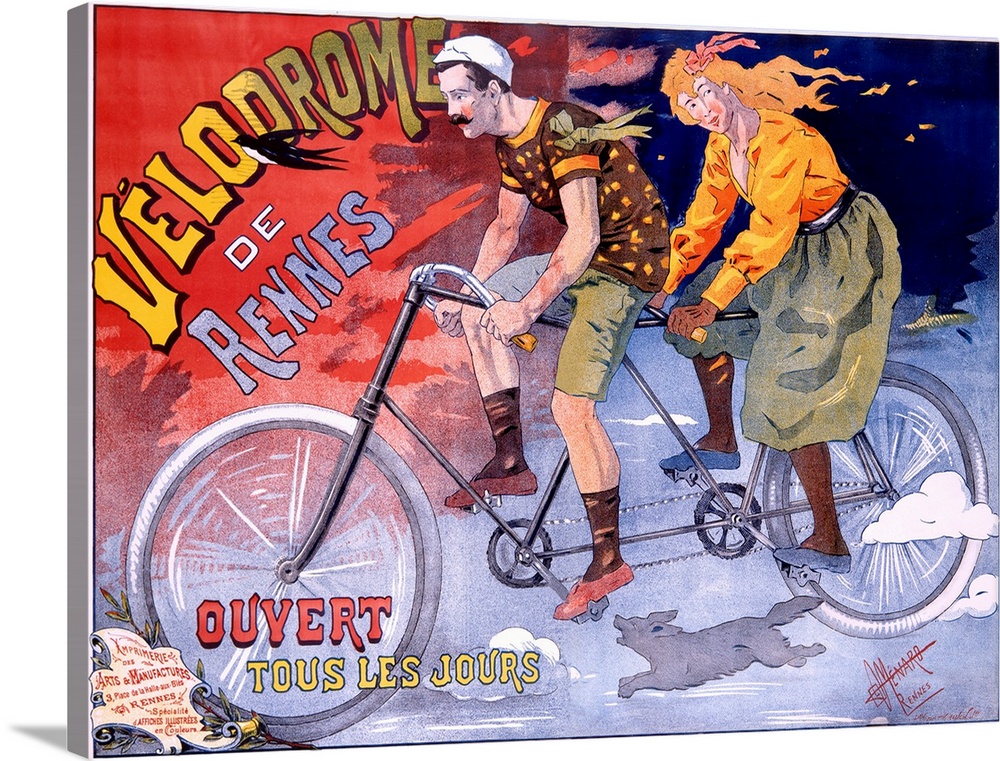The image is a hand-drawn, cartoonish-style illustration that serves as either a movie poster or a book cover. It prominently features two characters riding a tandem bicycle from right to left, with clouds depicted around the tires to give a sense of movement. The man in the front is wearing a white cap, colorful clothes including light green shorts, brown socks, red shoes, a brown and orange t-shirt, and has a black mustache. The woman behind him is wearing a long green skirt, brown leggings, blue shoes, a long-sleeved orange blouse, brown gloves, and has orange hair flowing behind her, indicating the wind. Their vibrant attire includes shades of brown, orange, green, red, yellow, and blue, with some gray and black. Accompanying them is a small gray dog running beneath the bike. The text "Vellumor Direns" is visible on the left side of the image. The woman gazes towards the viewer, while the man looks straight ahead. The artistic overlay appears three-dimensional, almost popping out from the wall.